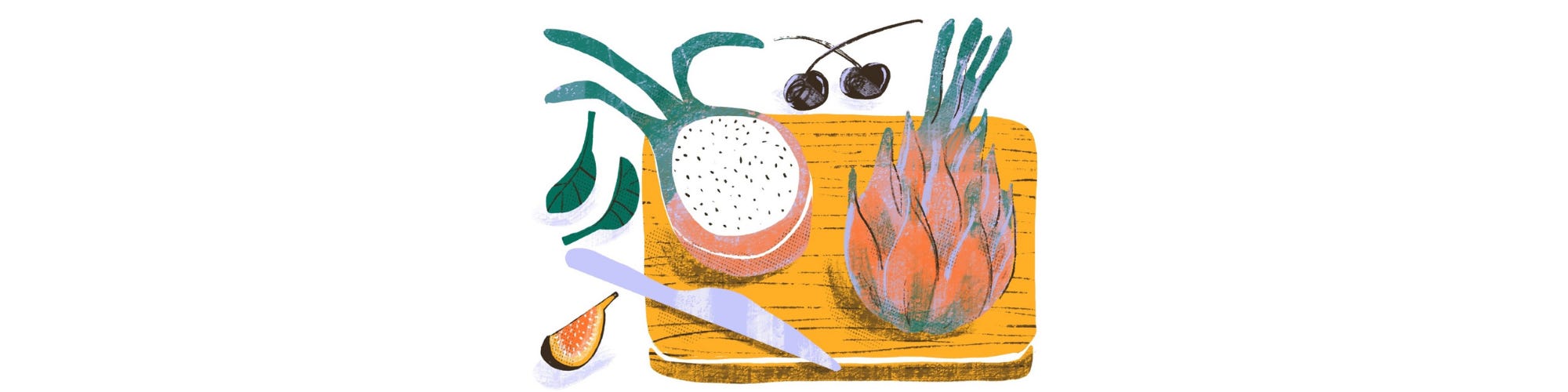This digitally created image features a wooden chopping board with a yellow-brown hue. Central to the composition is a detailed depiction of a dragon fruit. The fruit has a distinctive spiky, reddish-orange rind with green stems. One whole dragon fruit is placed beside a halved one, revealing its bright white interior speckled with black seeds, a telltale sign of the tropical fruit. Positioned near the cutting board are two black cherries with stems, a silver knife, and clusters of green leaves, adding to the vibrant yet slightly off-color aesthetic. The background is predominantly white, enhancing the colorful elements of the artwork.